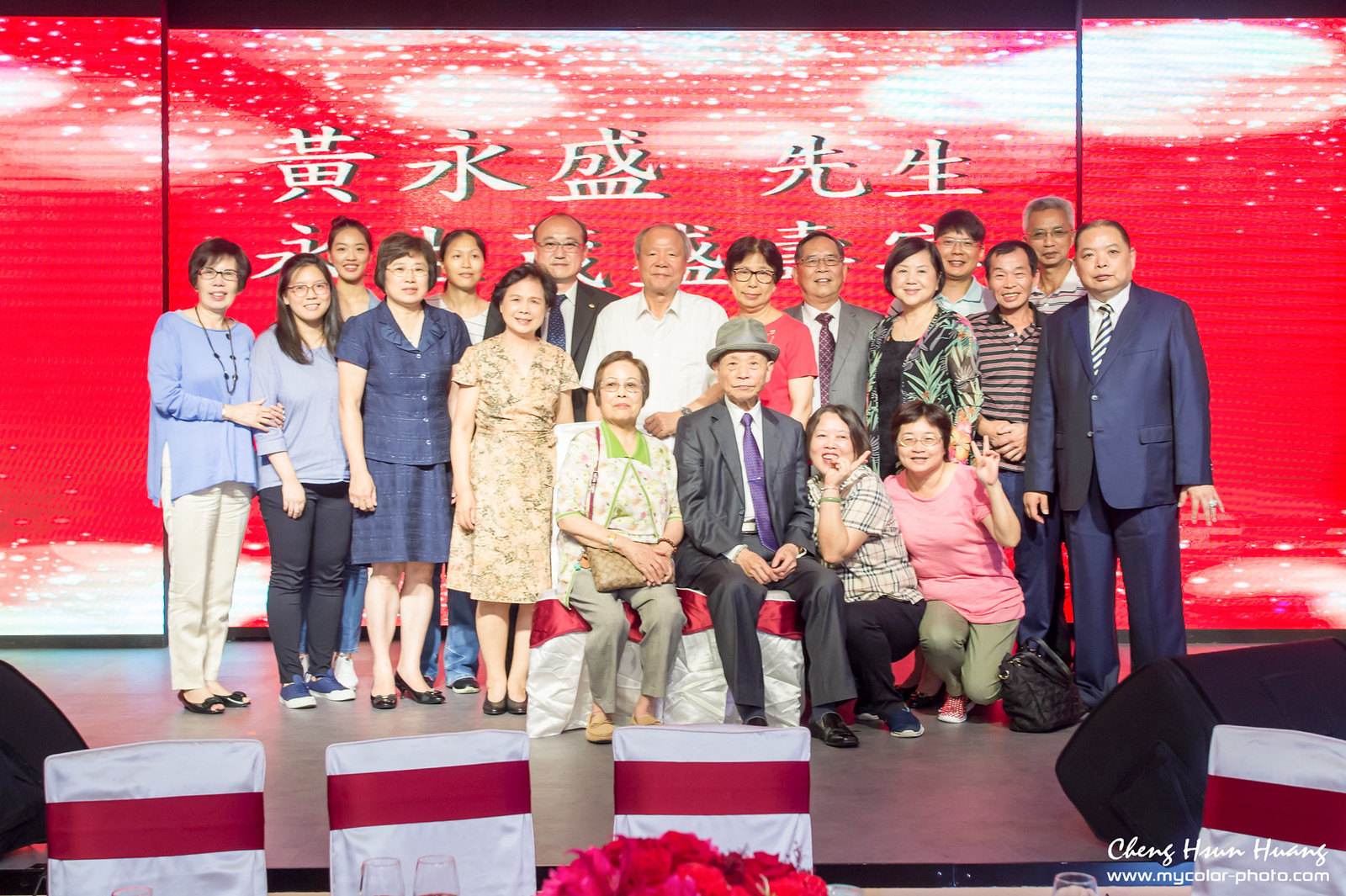This photograph captures a group of 20 to 25 people of Chinese ethnicity posed on an indoor stage. The group, consisting of mostly middle-aged or older individuals, includes both men and women, with women predominantly on the left and men on the right. Two older individuals are seated on chairs at the front, flanked by two women kneeling or crouched beside them, while the rest are standing behind in a formal yet casual arrangement. All members of the group are smiling, adding to the overall warm and celebratory atmosphere of the scene.

The backdrop features a large red display screen or wall with Chinese text, accented by white details, giving the impression of a formal event or celebration. In front of the group, four chairs, partially visible, are adorned with white covers and red bows, reminiscent of a reception setting. Additionally, flowers are visible at the lower part of the image, contributing to the decorative ambiance. The bottom right corner of the image contains the text "Cheng Huan Wang www.mycolor-photo.com," attributing the photograph to the specified photographer.